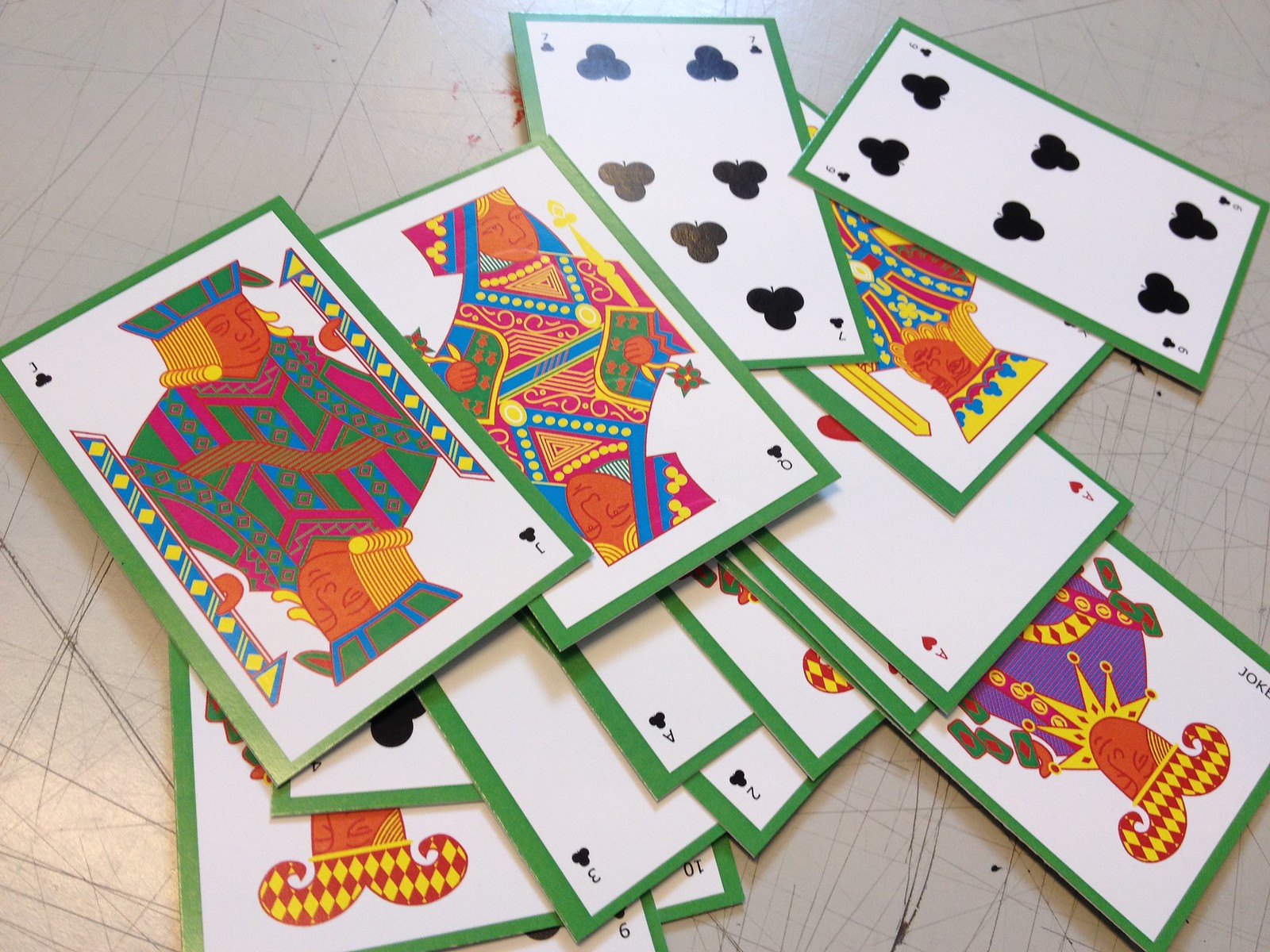The image showcases a scattered pile of playing cards resting on a white surface, visibly marred by numerous scratches running in various directions. The cards' design features a distinct green border on a white background. The topmost card is a Jack of Clubs, partially overlaying a Queen of Clubs. The vibrant colors of the cards—dark green, pink, blue, brown, and yellow—stand out strikingly. Among the scattered cards, a Joker, an Ace of Hearts, an Ace of Clubs, a Three of Clubs, a Two of Clubs, a Six of Clubs, and a Seven of Clubs are also discernible. The overall scene is a vivid display of playing cards amidst a well-worn and textured surface.